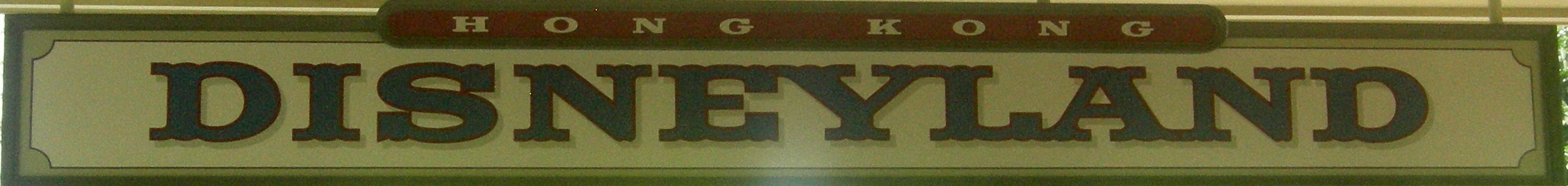In this image, we see a cropped section of a sign prominently featuring the text "Hong Kong Disneyland." The sign's design includes a red background at the top with the words "Hong Kong" in bold white block letters. Below this, the word "Disneyland" is displayed on a white background with a gray border, presented in green letters. The entire sign is framed by a green border and appears to be suspended from a pole, with mounting supports visibly attaching the sign to either side of the pole.